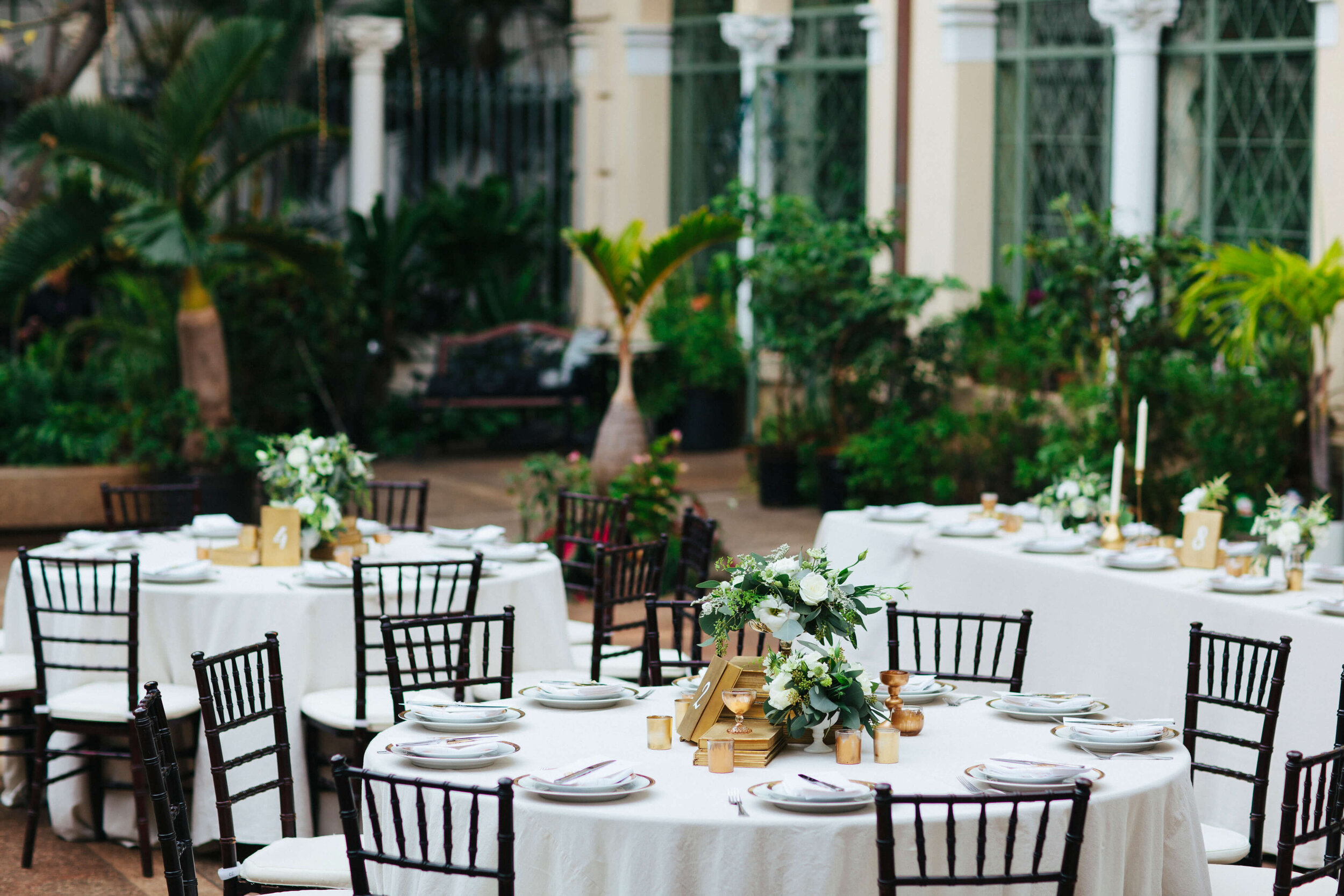The photograph depicts a sophisticated wedding reception scene set against a lush, tropical backdrop, evoking an elegant and serene atmosphere. In the foreground, two large, round tables draped with pristine white tablecloths are surrounded by approximately eight dark-colored, possibly black, chairs. These tables are meticulously arranged with plates, silverware, and delicate white floral centerpieces, complemented by candles and golden decorations. One table prominently displays the number two in a white numeral, while another table in the background is marked with the number four.

Positioned slightly to the right is a rectangular table, likely reserved for the bride and groom. This table, similar in decoration to the round tables, is labeled number eight and features additional intricate place settings. The scene is enveloped in tropical greenery, with ferns, palm trees, and various other lush plants creating a verdant backdrop. Some elements, such as green slatted windows and white columns, suggest this setting could be either an outdoor garden or an indoor greenhouse-like venue. Additional details, like a bench and tropical plants, enhance the patio environment ambiance. The tables in the foreground are in sharp focus, while the background elements appear slightly blurred, emphasizing the intimate and elegant setup of the wedding reception.